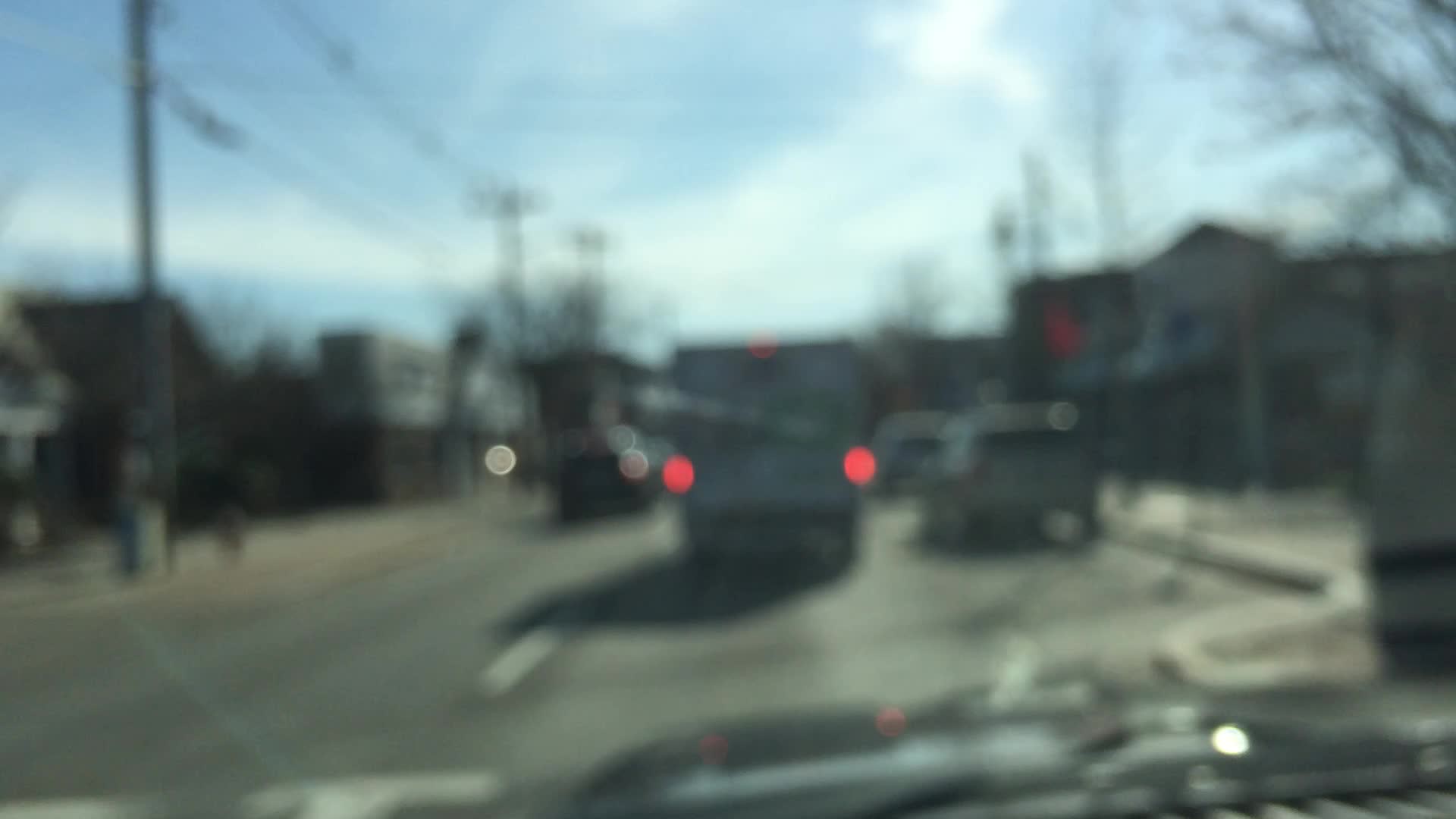The photograph, though very blurry, captures the point of view from a car windshield on a bright, sunny day, with blue skies and white clouds. The scene appears to take place in a small town or residential area that also includes various stores and commercial establishments. Visible from the windshield, there's a large tractor trailer directly ahead, noticeable by its prominent red brake lights. To the left, you can discern electrical poles and wires stretching overhead along with some houses and commercial buildings, including what seems to be a brick storefront. On the far left, there's a large train or trolley on the third lane. On the right side, cars are parked along the street near some shops, perhaps in a metered parking area, and there are trees with bare branches, suggesting it's either fall or winter. The clarity is compromised by glares and the general blurriness of the photo.